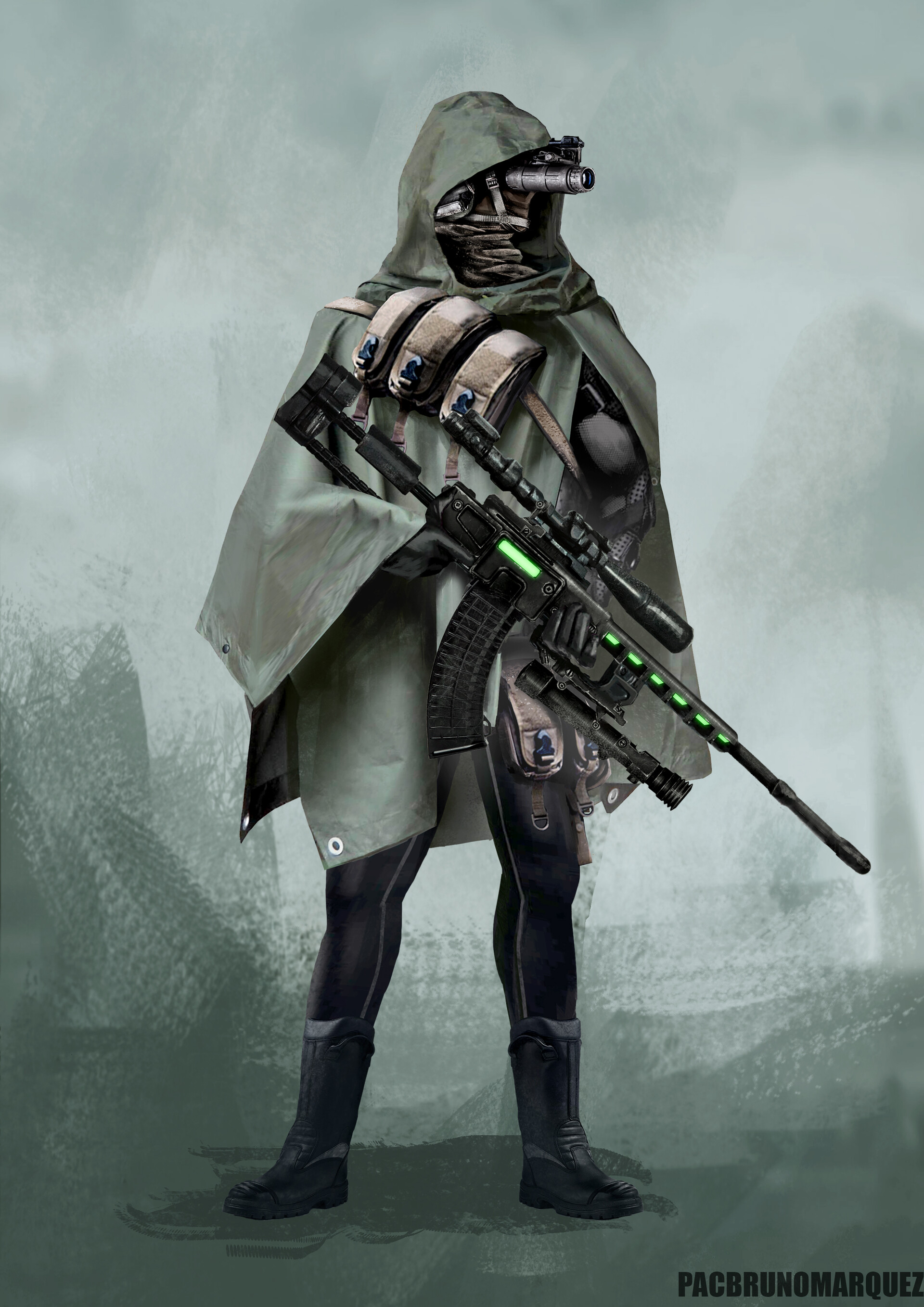This detailed image showcases a futuristic soldier with a complex array of equipment, set against a dynamic backdrop. The background features a green gradient with a cloudy upper section that transitions into a dark, navy-green, painted-like floor at the bottom. The soldier, adorned in a dark green hooded shawl reminiscent of a rainproof poncho, reveals robotic elements through a spring-like structure beneath its neck. The face is masked and features a large camera-like device emanating from its eye. The soldier wears black boots and dark black legging trousers, accented by thin, long gray stripes. Over its shoulder, it has a strap fitted with three brown satchel or magazine pouches.

The soldier clutches an imposing black sniper rifle with neon green accents and a large scope. This rifle is equipped with an extended buttstock, a large barrel, and a prominent ammunition magazine, appearing more sizable than the soldier itself. Small neon green lights embellish the neck of the gun, accompanied by another green light near the top, just above the ammunition. The scene suggests an artwork of a militarized, possibly video game character, offering a blend of advanced technology and tactical gear. The image is copyrighted by Pac Bruno Marquez, as indicated in black lettering at the bottom right corner.